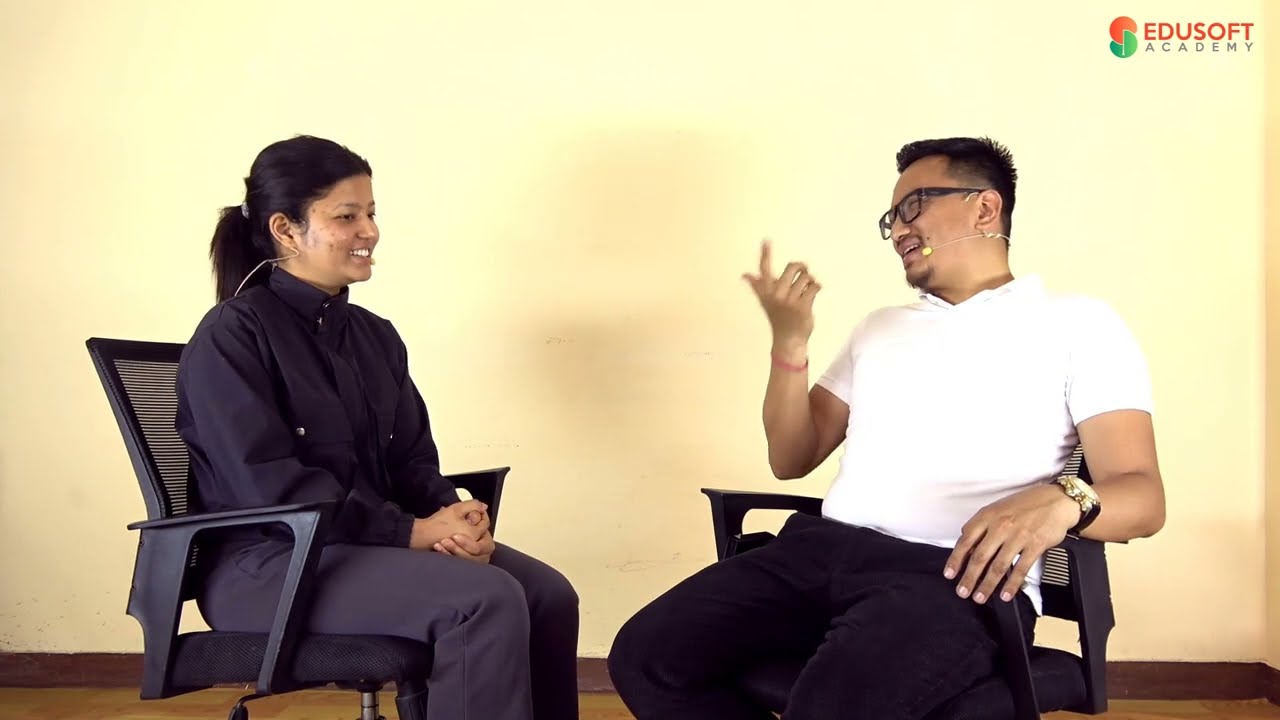In the image, we have a man and a woman sitting in comfortable black chairs, engaged in what appears to be an interview or podcast, given their use of microphones. The setting is indoors with an off-white, soft yellow, or peach-colored wall in the background and a light brown floor. The woman, positioned on the left, has medium darker-toned skin, black hair in a ponytail, and dark eyebrows. She is leaning slightly forward with a smile, wearing a navy blue jacket or a black long-sleeve button-up shirt and dark gray or black pants. Her hands are clasped in front of her lap. The man, positioned on the right, has darker skin, short black hair that's shaved on the sides and spiked on top, and a short black goatee. He is wearing thick black plastic-rimmed glasses, a white pullover collared shirt, and black pants. He has a gold watch with a black band on his left wrist and a red band on his right wrist. He is leaning back in his chair, pointing his index finger towards the ceiling with his right hand. Positioned centrally, they appear to be in a casual yet intimate setting, likely part of a presentation or interview as suggested by the "Edusoft Academy" logo in the top right corner. The image features various colors, including different shades of brown, off-white, black, white, gray, red, and green.